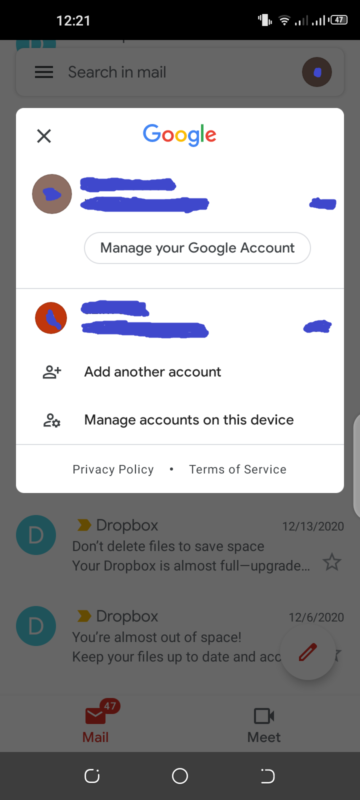The image depicts a screenshot taken on a cell phone. At the top of the image, a black header shows the phone's status bar which includes the current time on the left side. Moving rightwards, various icons are visible: sound settings indicating the phone is on vibrate, followed by a Wi-Fi signal meter, a battery level indicator, and network signal strength.

Dominating the screen is a white pop-up box labeled "Google," with personal information crossed out for privacy. The pop-up features several options: "Manage your Google Account," "Add another account," and "Manage accounts on this device." Below the pop-up, part of a search bar reads "Search in mail," suggesting that the screenshot was taken from within an email application.

Near the bottom of the screen, a notification from Dropbox warns, "Don't delete files to save space. Your Dropbox is almost full." Additionally, it stresses, "Dropbox, you're almost out of space. Keep your files up to date."

The combination of these elements provides a comprehensive glimpse into the user’s phone interface at the moment the screenshot was taken.